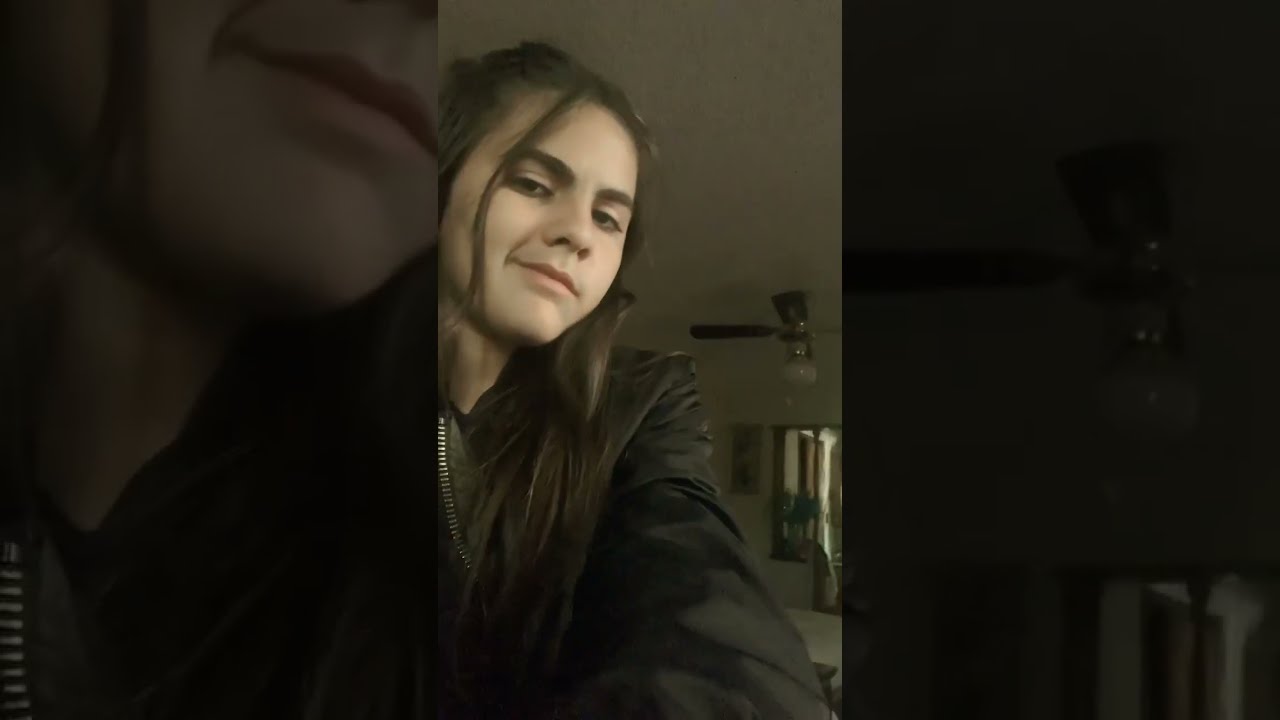The image shows a young girl with fair skin, characterized by her thick brown eyebrows and very long dark brown hair, which is mostly pulled back except for a single strand that falls over her right eye. She is wearing a black jacket with a zipper and is slightly smirking while taking a selfie. The background features white walls, a ceiling fan, and possibly a kitchen counter with a small mirror or light on it. The photo itself, in high definition, is centered and bordered by blurred, close-up portions of the main image, creating a focused effect. There are steps or perhaps a walkway visible in the background, adding depth to the domestic setting.